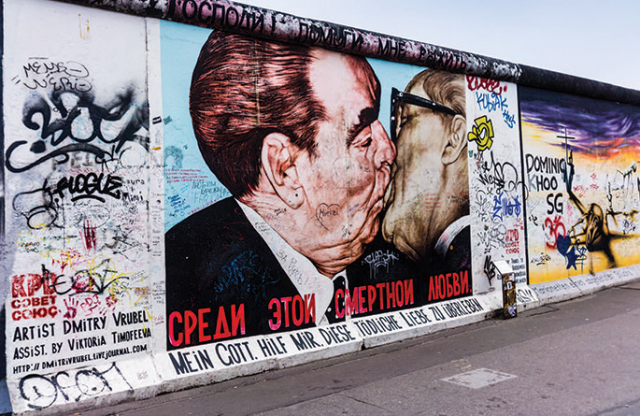This image captures a vibrant graffiti wall, likely located in a foreign country that could be Russia. The focal point of the mural is an artistic depiction of a white man in a black jacket and white shirt, sharing a kiss with an older white gentleman wearing glasses. This striking piece, perhaps a social or political statement, is credited to an artist named Dimitri, though his full name is not entirely legible. Adjacent to this central image is another, less refined piece of graffiti, featuring the text "DOMINO HOLE SG" and what appears to be an octopus. The wall as a whole is a vivid canvas of public expression, blending detailed artwork with raw street art elements.